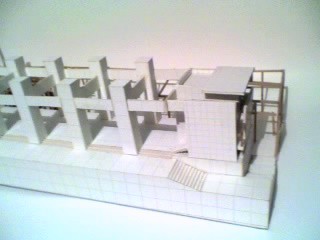The image features a highly detailed computer-generated rendering of a miniature architectural model, captured indoors against a predominantly white backdrop. The model, meticulously constructed from square-shaped cubes arranged in rows, depicts an unfinished building structure. On the left side, numerous vertical square poles are interconnected by horizontal support beams. The right side showcases a more defined rectangular structure with an elevated roof, surrounded by walls. Leading up to this building, there’s a miniature staircase consisting of approximately ten steps, which connects to a small runway, with an extended runway beside it. This intricate model, characterized by straight lines and geometric forms, conveys a scene of architectural development, complete with exposed floors and beams, reflecting a stage just before construction completion.